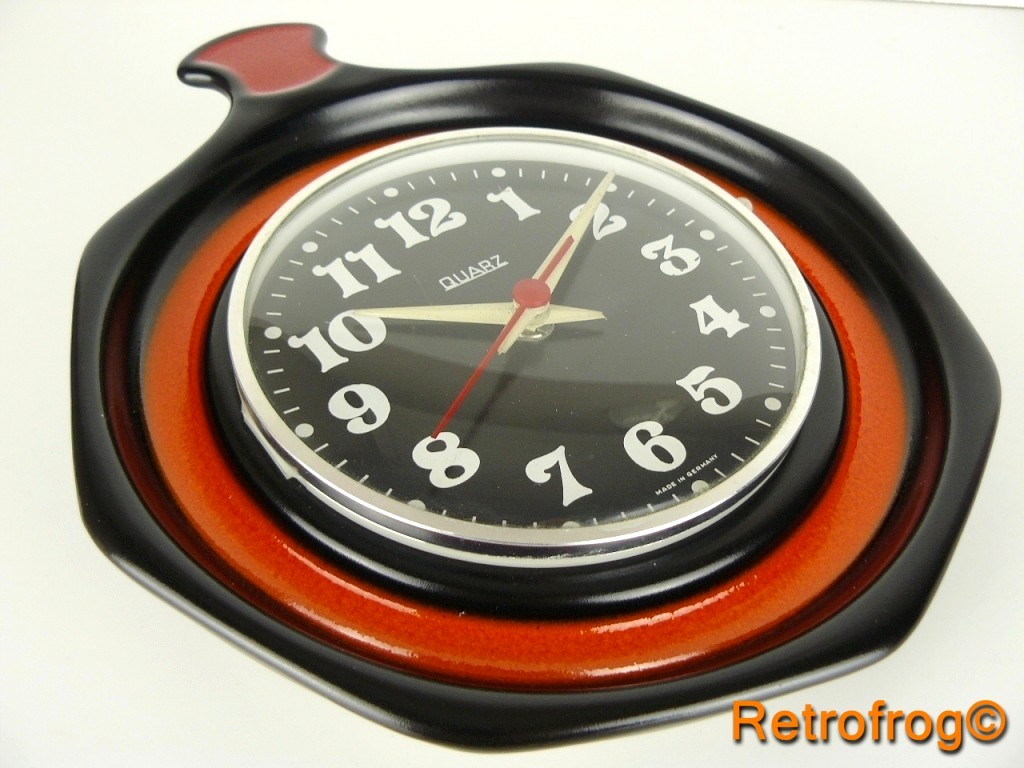This image features a clock displayed laying on its back and rotated approximately to the 11 o'clock position from the upper left to the lower right side of the frame. The clock has a distinctive appearance, crafted from plastic and housed in an octagonal, rounded black frame with an inner red ring. Its striking design is further highlighted by the black center housing. The clock face is black, showcasing bold white numbers and traditional white hour and minute hands, complemented by a vibrant red second hand. It operates on a quartz movement. In the lower right corner of the image, against an off-white background, "Retro Frog" is inscribed in orange letters, accompanied by a copyright symbol. Additionally, the clock bears a mark of craftsmanship, proudly stating that it was made in Germany.